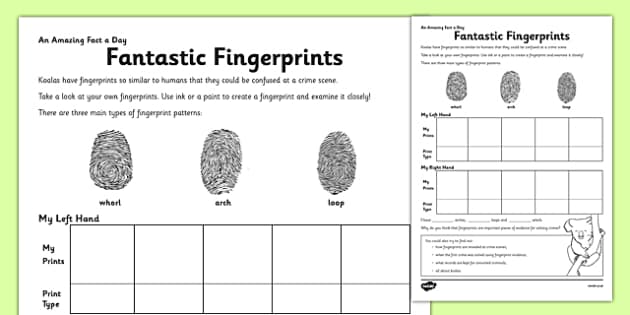The image depicts a children’s educational fingerprint activity sheet, titled "Fantastic Fingerprints," set on a lime green background with white and black text. The sheet appears twice: a zoomed-in view on the left and a smaller, full-page view on the right. The top of the document features the heading "An Amazing Fact a Day: Fantastic Fingerprints," accompanied by a fascinating fact: "Koalas have fingerprints so similar to humans that they could be confused at a crime scene." Below the text are illustrations of three fingerprint patterns—whorl, arch, and loop—each labeled accordingly. The sheet provides a grid labeled "My Left Hand," "My Prints," and "Print Type" with boxes for users to imprint their own fingerprints, using ink or paint, for comparison. Additionally, a line drawing of a koala holding a branch is sketched in the bottom right corner, and there is a faint watermark on the bottom left. The layout suggests this sheet is a downloadable or purchasable activity designed to engage children in learning about fingerprint patterns.